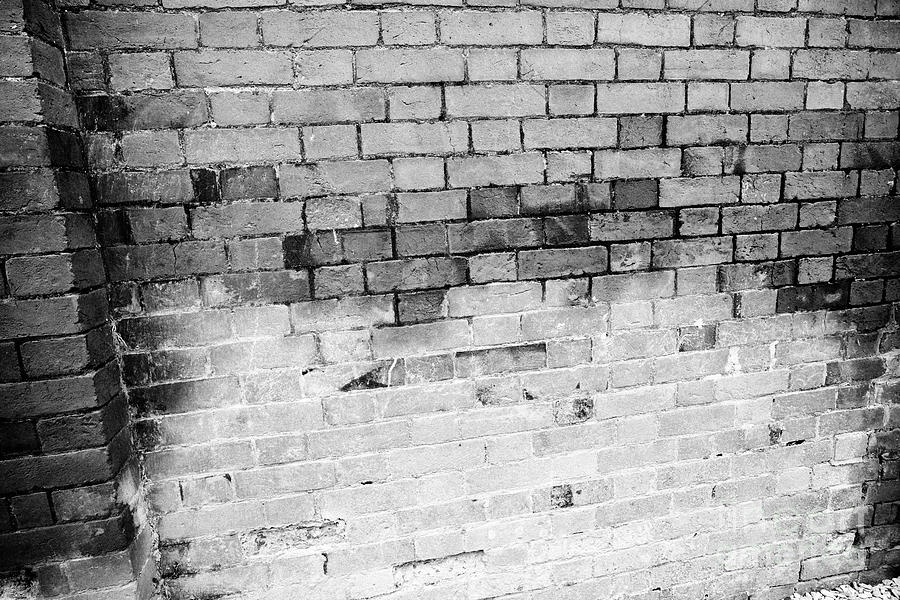In this black and white photograph, we see a brick wall that appears to be either under construction or in a state of disrepair. The wall stands at an estimated height of six feet or higher and features bricks of varying shades, with lighter and darker bricks intermixed. The bottom half of the wall is notably different, covered in a white substance that resembles powder or primer, not paint. This section of the wall shows significant wear and damage: many bricks are cracked, scratched, or partially missing, and the mortar between them is scant, exposing gaps that suggest a crumbling structure. The upper portion of the wall appears more intact but still shows signs of age and weather, with some bricks appearing water-stained. On the left side, there is a protruding section resembling a pillar, extending about eight inches further than the rest of the wall. This detailed image captures the wall's varying conditions, from the almost powdery, damaged lower section to the somewhat sturdier but still weathered upper area.